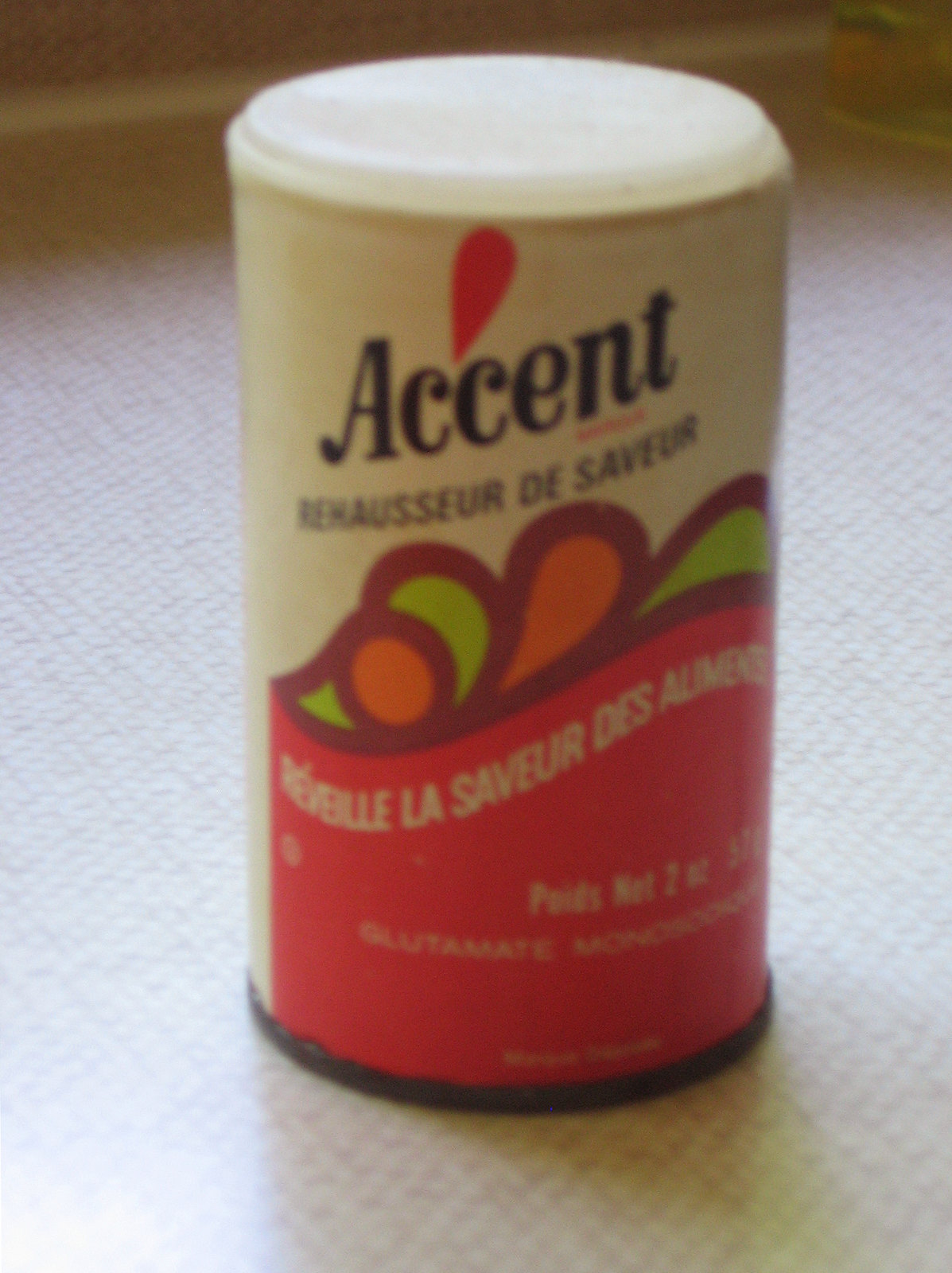This color photograph captures a slightly blurry image of a small, predominantly white canister labeled "Accent," which is resting on a carpeted floor or possibly a white countertop. The canister, which appears to contain some type of seasoning, has a distinctive red band along its bottom half and features a combination of green and orange wavy patterns as part of the decorative design. The label includes the word "Accent" in bold, black letters, along with additional French text that reads "Rehausser de Saveur," and further French text in a pink section at the bottom. The canister is marked with a net weight of two ounces (57 grams). This particular product might contain monosodium glutamate, as suggested by some readable portions of the text.